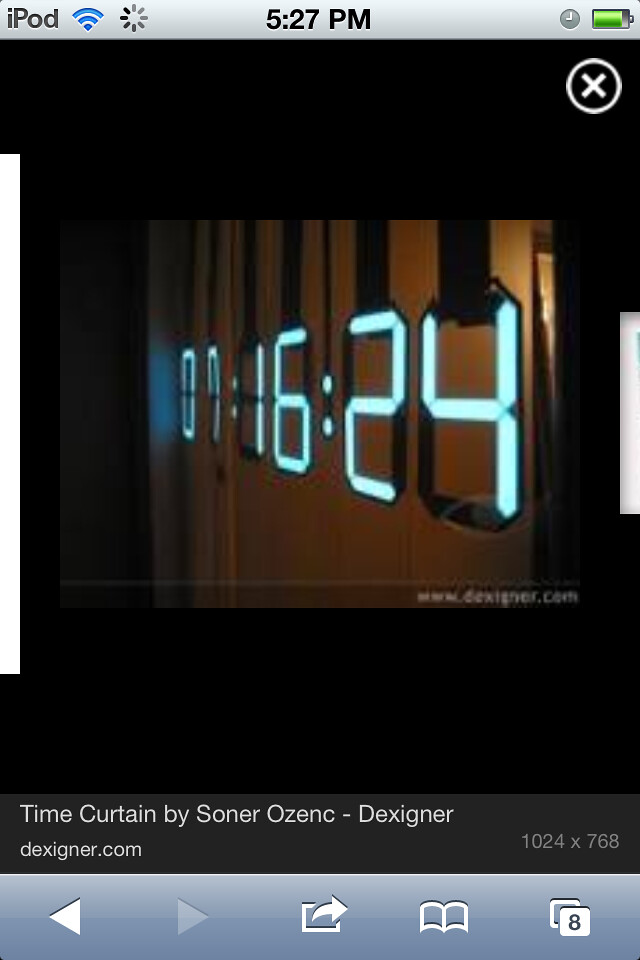This image is a screenshot of an iPod displaying a digital clock interface. In the center, angled slightly from the side, bright blue neon numbers read "07:16:24," indicating the time in hours, minutes, and seconds against a muted white background with black lines resembling piano keys. The top of the screen features a gray strip with "iPod" in black, followed by the Wi-Fi signal, a starburst symbol, the time "5:27 p.m.," a clock hand icon, and the battery level indicator in green. At the bottom, text in a blue-gray rectangle reads "Time Curtain by Soner Ozenk," with an adjacent white arrow pointing left, a grayed-out right arrow, a book icon, and squares marked with "8." The overall appearance of the display, designed by Soner Ozenk and described as a "Time Curtain," suggests a modern, potentially futuristic aesthetic.